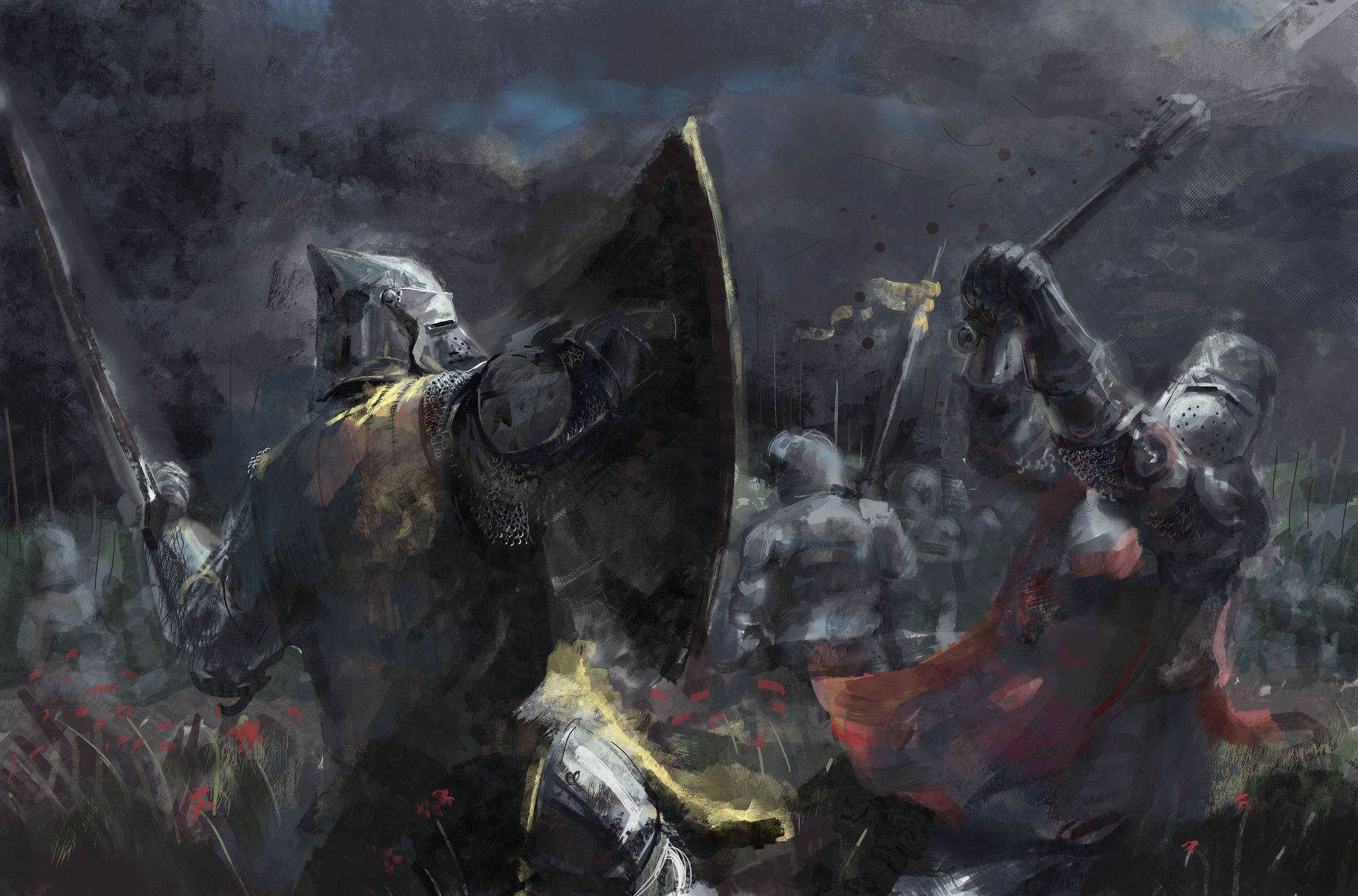This detailed painting illustrates a dramatic battle scene from the medieval era. The foreground features two armored men engaged in intense combat. The warrior on the left wields a sword in his left hand and a large shield in his right. The other soldier, positioned to the right, appears to be striking at him with a weapon. Both warriors are clad in full metal armor covering their heads and bodies, reinforcing the historical setting of the Middle Ages. The ground is dotted with splotches of red flowers, adding a stark contrast against the dark, ominous sky filled with predominantly gray clouds. However, patches of blue sky peek through, lending a glimmer of hope in the otherwise foreboding atmosphere. In the background, more armored fighters can be seen, along with a distinct yellow flag. Despite the vivid details rendered by the artist, there is no clear identifying information such as the name of the battle or the location. The painting is likely signed by the artist at the bottom, although the signature is not visible in the image.